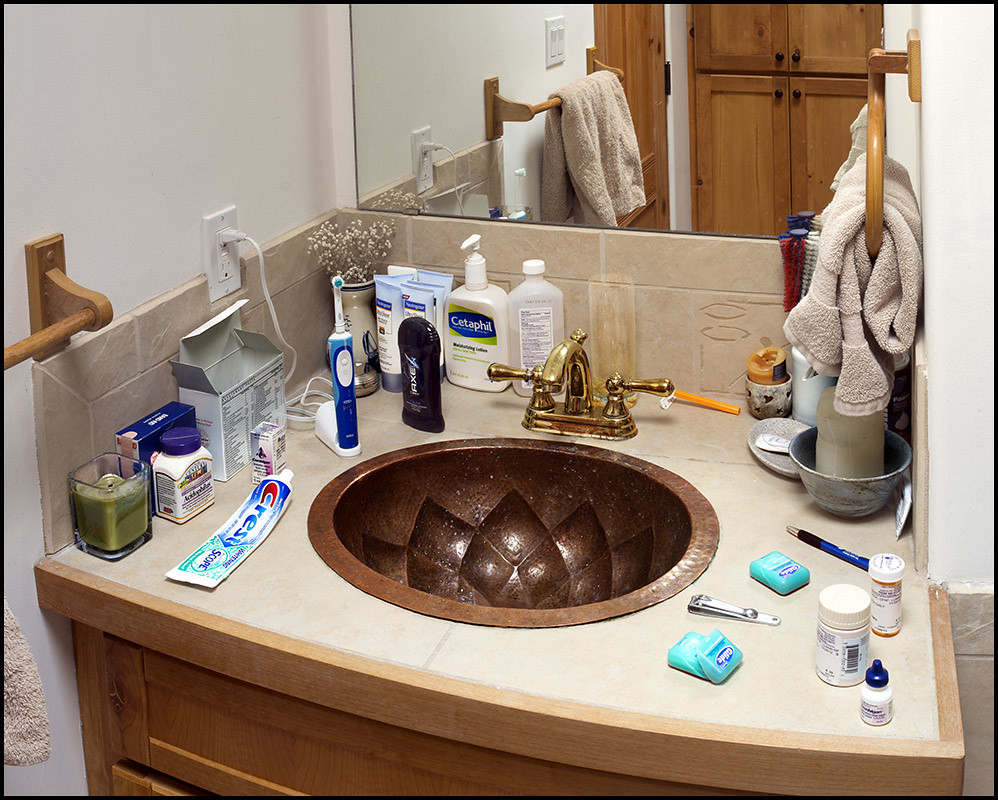In this photorealistic image, a bathroom sink is captured with a distorted fisheye lens effect, causing the edges of the picture to appear bent. The countertop boasts a very tan color, juxtaposed with a wood-finished edging. Central to the scene stands a gold-colored, possibly brass, faucet over a dark brown, marble-patterned sink. 

Arrayed around the sink are various personal care items: a tube of Crest toothpaste, a blue electric toothbrush with its cord plugged into a nearby electric outlet, and an Axe roll-on deodorant. The setup also includes containers of Cetaphil lotion, an assortment of small Neutrogena containers in blue and white, and a white vase with small yellow plants to the left.

On the bottom left corner of the countertop, one can spot a candle, a small white vitamin bottle with a purple top, and a blue Band-Aid box. On the other side, there's a collection of dental floss containers in white and blue, a nail clipper, and some pill medication bottles. This meticulously detailed arrangement of everyday items situates the viewer intimately within a familiar, yet uniquely stylized, setting.